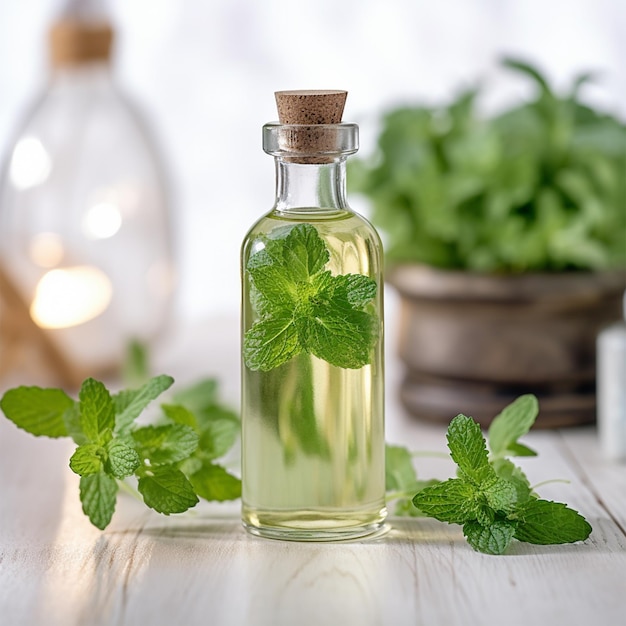The image features a small glass vial with a dark brown cork stopper, almost filled to the top with a yellowish-green liquid. Suspended within the liquid is a mint leaf with five distinct lobes. Flanking the vial on either side are additional mint leaves, each also displaying five separate lobes, resting on a light-gray, whitewashed wooden table that showcases its grain patterns. In the blurred background, to the left stands a larger clear-glass jug, and to the right, a brown wooden pot houses a lush, vibrant mint plant, indicating the source of the leaves both in and around the vial. The scene exudes a rustic, herbal essence with a focus on natural elements.